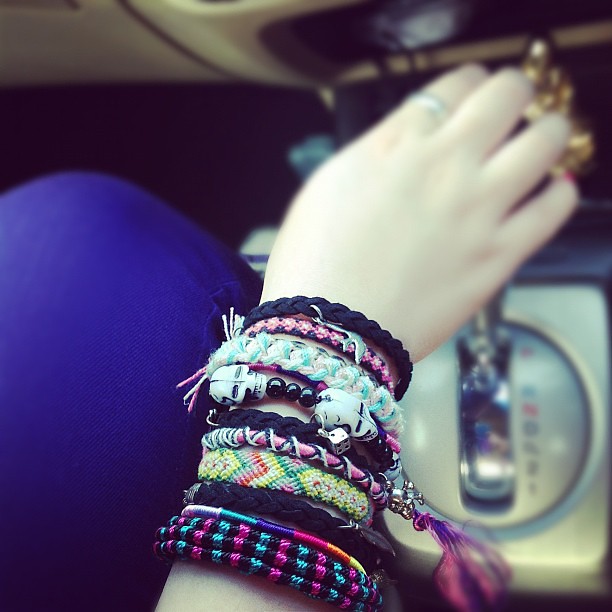This is an indoor color photograph taken from above that focuses on a young woman's forearm and hand resting on a gear shift in a car with a cream-colored interior. The image prominently features her arm adorned with a variety of colorful bracelets. These bracelets, approximately seven or eight in number, vary in material and design, including those with black and pink stripes, a rainbow of colors, and combinations of yellow, green, red, and pink. Some bracelets are beaded, some have little charms, and others are made of threads or wires. A ring is visible on the index finger of her right hand, which is somewhat out of focus. Her fingernails are painted pink, noticeable on her left pinky. Her left leg, clad in blue pants, is visible along the left side of the frame, while a bit of the car's front panel appears in the upper portion. The focal point of the photograph, however, remains the assorted bracelets on the woman’s wrist.